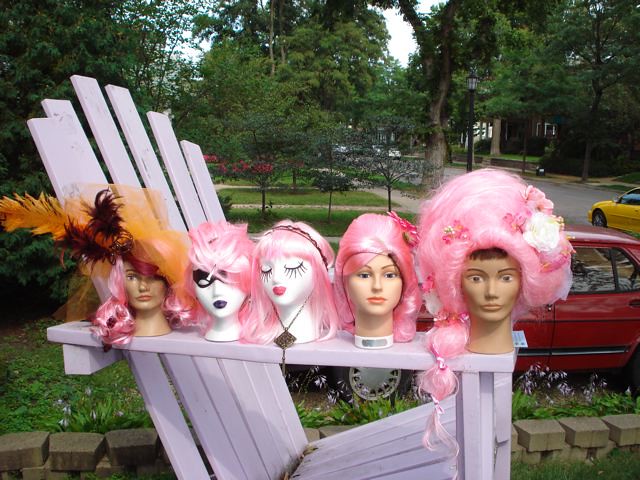In this outdoor photograph, we see a large white wooden lounge chair with slatted design, slightly tilted back with a fanned-out top, located in a shaded yard. The yard is framed by large overhanging trees and a small brick wall holding back lush vegetation, including some small purple flowers. Positioned along the right armrest of the chair are five distinct mannequin heads, each adorned with bright pink wigs styled differently. 

The first mannequin displays a large bouffant wig decorated with a big white flower, and has a brownish skin tone with natural makeup, appearing to look straight ahead with a surprised expression. The second mannequin has a somewhat tamer bouffant wig with flowers, featuring a peach-colored complexion and facing forward. The third mannequin sports a straight pink wig with bangs and a headband, painted white with closed eyes and long eyelashes, red lips, and wearing a black necklace. The fourth mannequin’s pink wig is messily styled; it’s painted white and has a black eye mask with black lipstick. The final mannequin's curly pink wig is accessorized with a big orange hat with feathers, and it has a peachy complexion with natural makeup.

In the background, there's a driveway with a red car parked and a street where a yellow car is driving, indicating this is the front of someone's house. The scene is shaded by large trees, with neighboring homes and lawns visible, adding to the suburban setting.